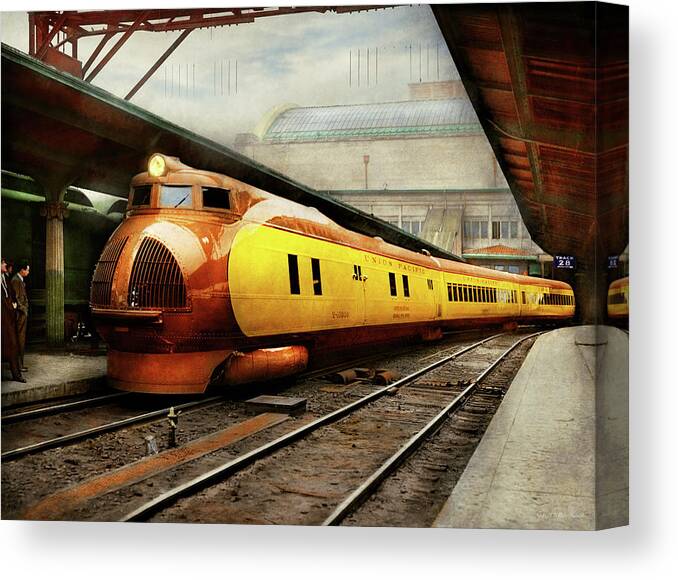This is a computer-generated image or painting of a futuristic, steampunk-inspired bullet train pulling up to a station. The train features a striking coppery-gold color with round, aerodynamic shaping, including a front adorned with vertical grates. The main body of the train is a deep brown-red color, transitioning to a school bus yellow on the windowed sides. The concrete platform it approaches is partially covered to protect passengers from the elements. Next to the train, two men in suits stand waiting. The scene is set against a backdrop of an Art Deco-style concrete building, topped with a distinctive blue and green domed roof. The sky above is blue with clouds, but peculiar evenly spaced black lines are present, creating an unusual atmospheric detail. The rail tracks are dusty and rusty, enhancing the vintage-industrial aesthetic of the scene. The words "Union Pacific" can be faintly seen on the side of the train, further grounding the image in a rich historical context.